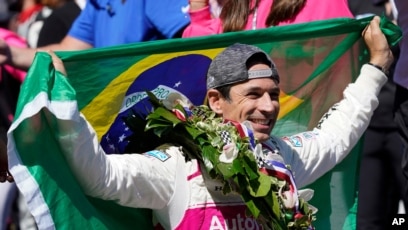The photograph captures a jubilant Brazilian athlete who has just won an event, likely a cycling or motorsport competition. Draped in a green Brazilian flag with a yellow and blue circle and white embroidery, he holds it triumphantly with both hands stretched wide. The athlete, dressed in a long white jacket adorned with various logos, wears a wreath made of flowers and leaves around his neck, with pink and light pink flowers and light green and dark green leaves. He also sports a backward baseball cap, revealing a glimpse of his black hair and a large smile. In the background, blurred spectators include a woman in a black shirt holding a red or pink garment, a man in a blue dress shirt, and a woman in a pink jacket, all cut off at the edges so their faces are not visible. The photo, taken during the day, bears the credit "AP" for Associated Press in the bottom right corner.